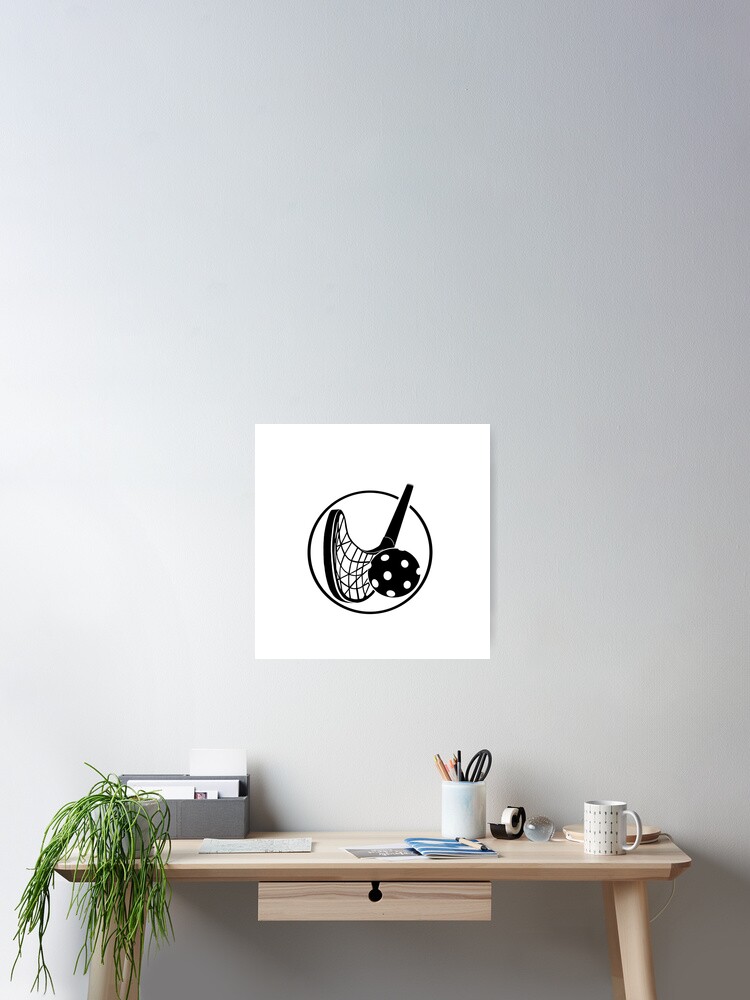The image depicts a small, subtle, wooden work desk situated against a light-colored wall, possibly white or light gray. On the wall in the background, there's a square piece of paper featuring a circle, a line, and images resembling a golf club and ball, or possibly a hockey stick and ball. The desk, light beige in color, is adorned with various items: a green plant hanging off the left side, a white lamp on the right, and a cup containing scissors and pencils. Additionally, there's a white coffee mug, a tape dispenser, some scattered papers and brochures, and a shallow drawer underneath the desk. The setup is completed with a piece on the left side of the desk for organizing paperwork.